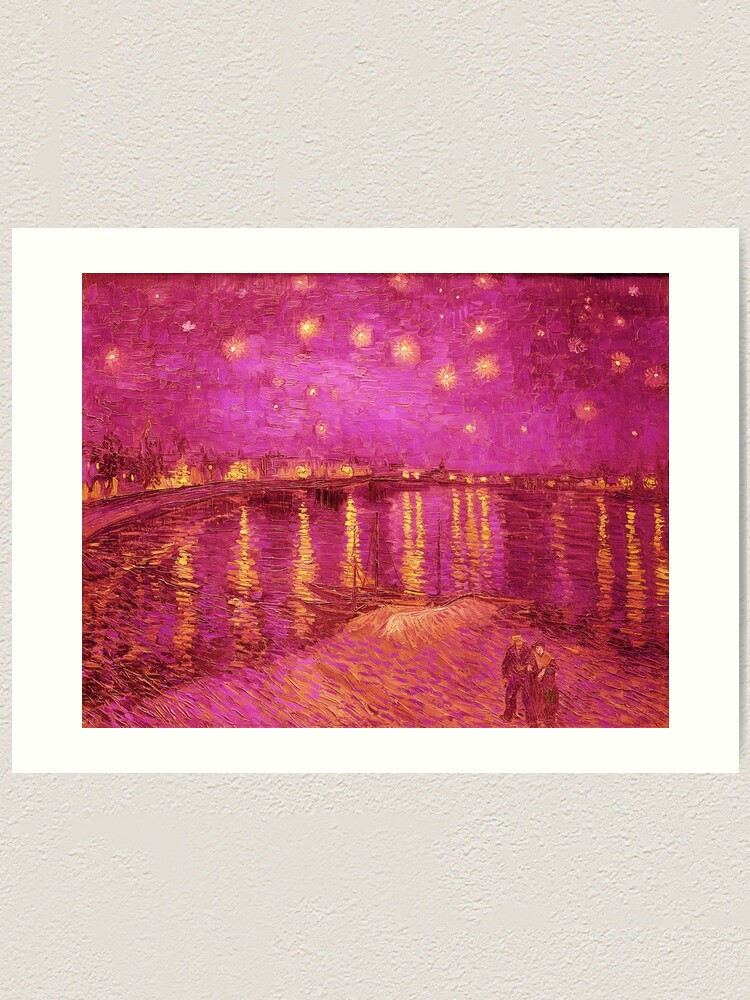The image depicts an elegant painting set within a white, matted border, mounted on a textured off-white wall. The art captures a vivid nightlife scene dominated by shades of pink, including fuchsia, magenta, hot pink, and light pink, with accents of yellow and gold. The sky is painted in various pink tones, adorned with golden stars. Along the horizon, darker pink buildings, resembling a cityscape, emit a warm, yellow glow which reflects off a pink-colored body of water below, creating striking vertical light patterns. Additionally, grassy areas in the foreground are painted in pinks and yellows. Near the bottom right corner, you see a dock with boats featuring masts, and a couple, possibly a man and a woman, colored in darker pink, is seen walking closely together. The painting, reminiscent of a Picasso style with bold colors applied using a palette knife, exudes a dreamy, watercolor-like quality.